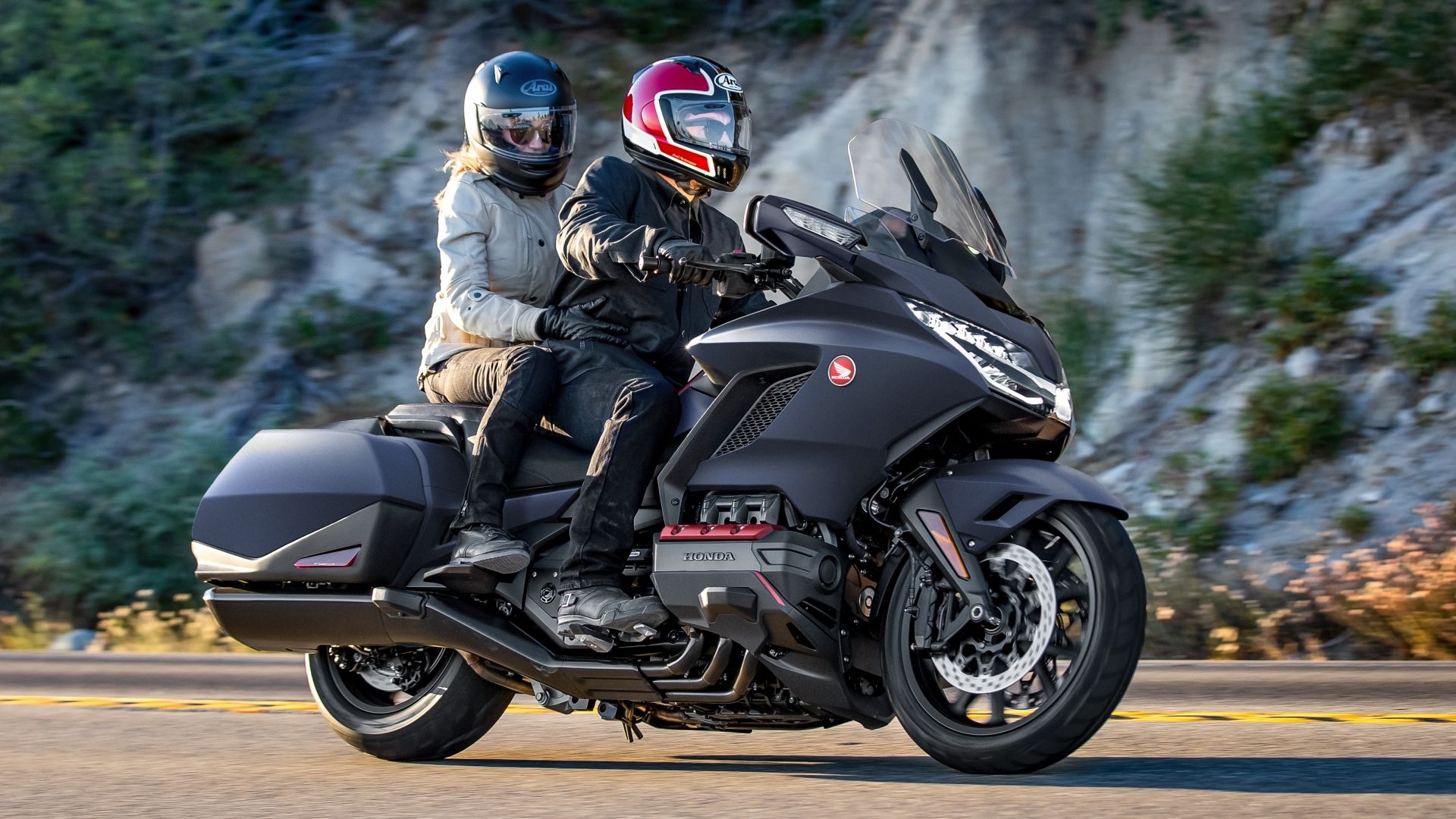This outdoor daytime photograph captures a Honda motorcycle with two riders traveling on a gray paved roadway marked by a solid yellow line down the center. The motorcycle, predominantly black with red accents on the engine and a red and white Honda insignia on the front, appears to be a large street bike, possibly a six-cylinder model with a large fairing and rear luggage fairings. The rider, a man at the controls, is dressed in a black leather jacket, black jeans, black leather boots, and a red, black, and white striped helmet, complemented by sunglasses. The passenger, a woman presumed to be his girlfriend or wife, clings to him while wearing a white leather jacket, black leather pants, black boots, a black full-face helmet, and sunglasses, with blondish hair visible at the back of her helmet.

In the background, the right side of the image is defined by a hillside or cliffside terrain composed of white stone and green foliage, along with some yellow plants and gray sandy areas. The sun illuminates parts of their outfits, lending a brown tint to the passenger's black pants. The rectangular photograph, roughly six inches wide and three inches high, is rich with detail, including the texture of the road and the surrounding natural landscape.